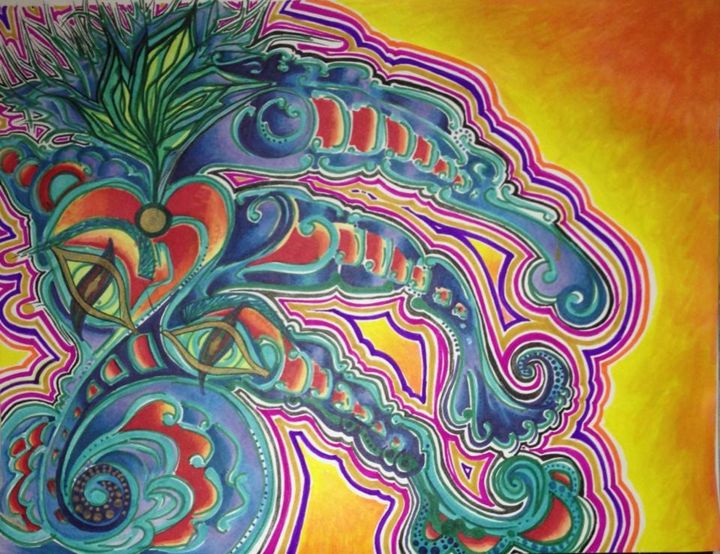This artwork is an abstract marker drawing exuding a vibrant 1960s hippie style, replete with swirls, paisleys, and human eyes. The image bursts with a multiplicity of bright colors including vivid reds, yellows, purples, magentas, and blues. The background features a radiant gradient, starting with a bright yellow at the center and gradually transitioning to a warm orange at the corners. There are intricate leaf imprints and designs interspersed throughout the artwork, adding to its whimsical nature. The drawing is characterized by a blob-like outline framed with a striped rainbow pattern, creating a striking contrast. Shading between some abstract sections adds depth and dimension to the colorful composition.